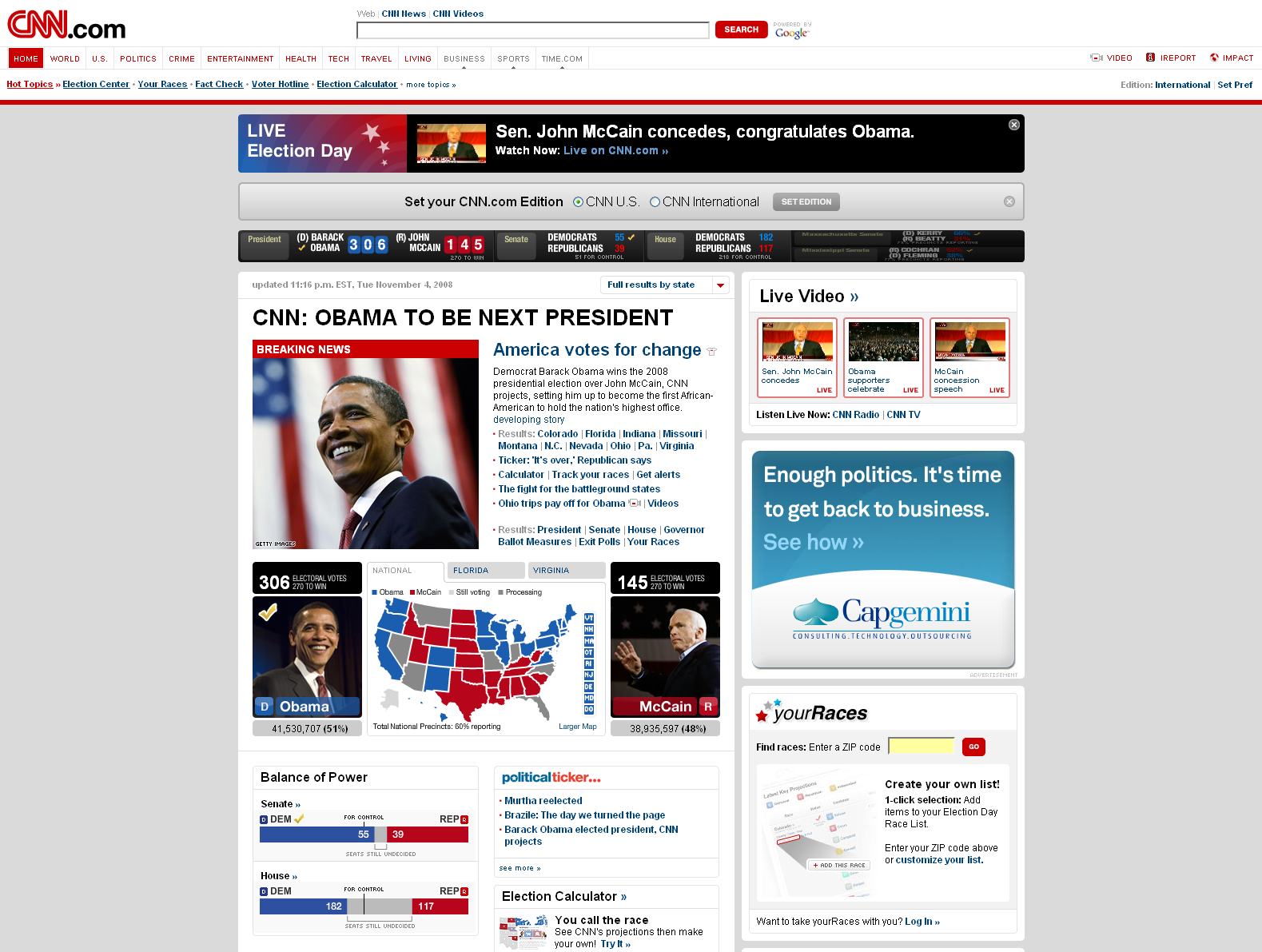This image captures the homepage of the CNN.com website during the historic 2008 Presidential Election. At the top of the page, although the text is small and difficult to read, the navigation and search bar are visible. Prominently displayed is the live coverage headline that reads, "Live Election Day." A breaking news banner announces, "John McCain concedes, congratulates Obama," followed by a "Watch Now" prompt. Below, a larger headline states, "Obama to be next president - Breaking News: America Votes for Change." The website reports that CNN projects Barack Obama as the winner of the 2008 Presidential Election over John McCain, setting Obama up to become the first African American to hold the national office. Accompanying the text are images of a triumphant Barack Obama.